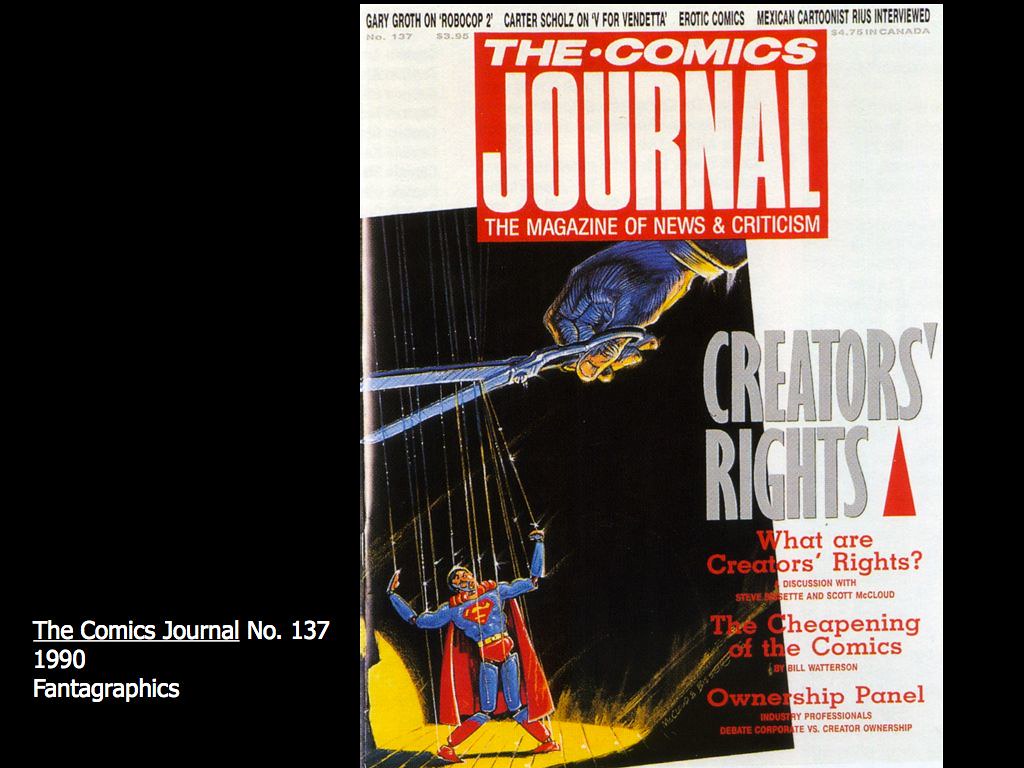This image depicts the cover of "The Comics Journal," a magazine focused on news and criticism in the comics industry. Set against a black background, the cover is positioned towards the center-right of the rectangular frame. In the bottom left corner of the image, text in white reads: "The Comics Journal, Number 137, 1990, Fantagraphics," arranged in three lines.

Dominating the cover is a vivid illustration of Superman depicted as a marionette, with strings attached to his limbs and body. His knees buckle under the tension, and a hand in the upper right corner threatens to sever the strings with a pair of scissors. The phrase "Creators' Rights" appears prominently on the right-hand side of the cover, with additional text asking, "What are Creators' Rights?" and discussing topics such as "The Cheapening of the Comics" and the "Ownership Panel," all rendered in red font.

At the top of the magazine, a red rectangle contains the title "The Comics Journal: The Magazine of News and Criticism," with the words appearing in descending order of font size, the largest being "Journal." In addition, the top also features smaller text highlighting articles within the issue, including Gary Groth on "Robocop 2," Carter Scholz on "V for Vendetta," as well as pieces on Erotic Comics and an interview with Mexican cartoonist Rius.